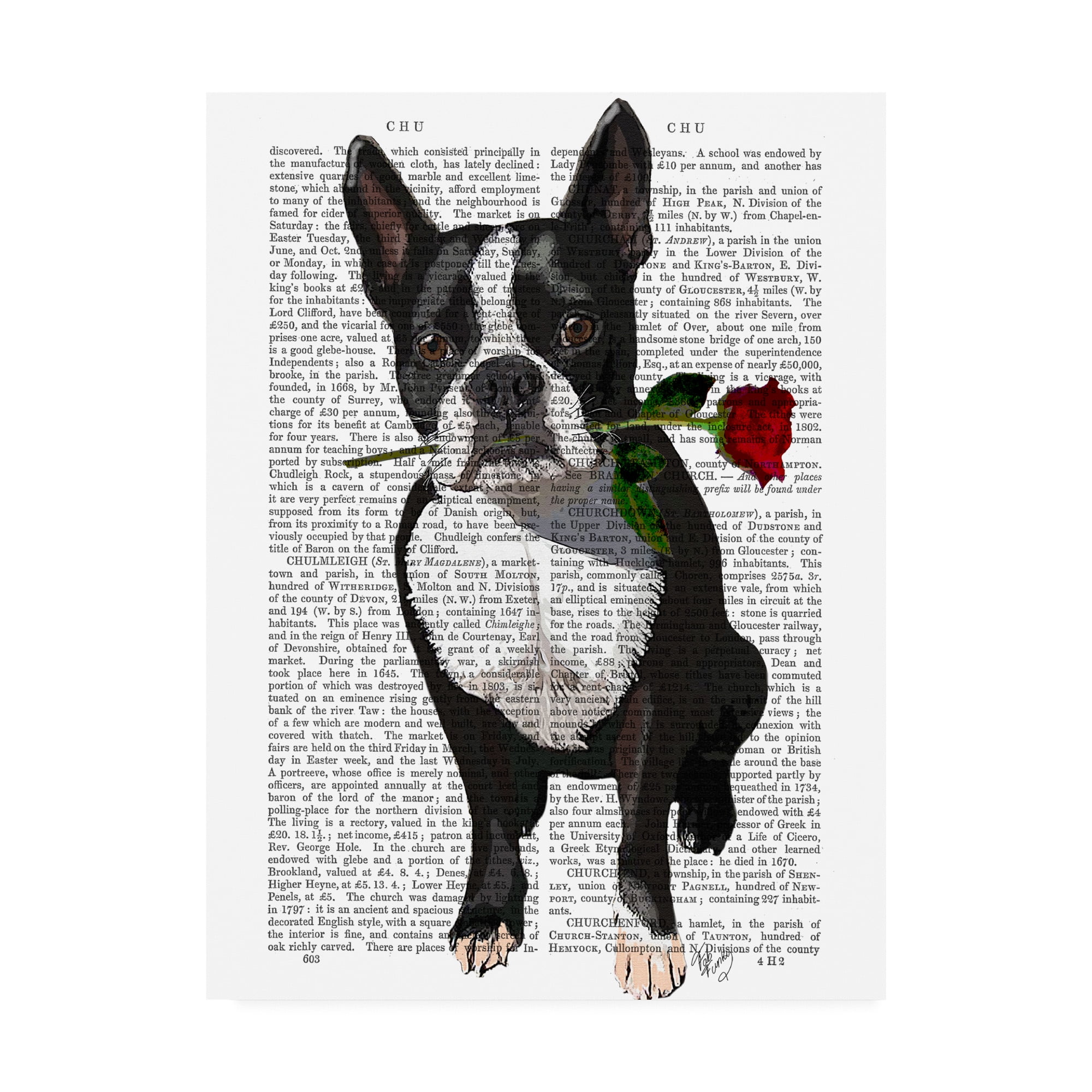The image depicts a page from a book written in English, featuring a small, adult dog that appears to blend into the text on the page. The dog, which has the distinctive features of a Boston Terrier, is seated and holds a red rose with green leaves in its mouth, leaning the flower on the left side of its face. Its fur is predominantly black, with white patches that are partly translucent, allowing the book's text to show through. The dog has brown eyes, ears that stand up with pink insides, and pinkish flesh-colored nails. Despite its somewhat innocent and sad expression, the animal's position and integration into the page text, which includes the word "Choo Choo" (spelled "C-H-U, C-H-U"), create a striking and surreal composition.